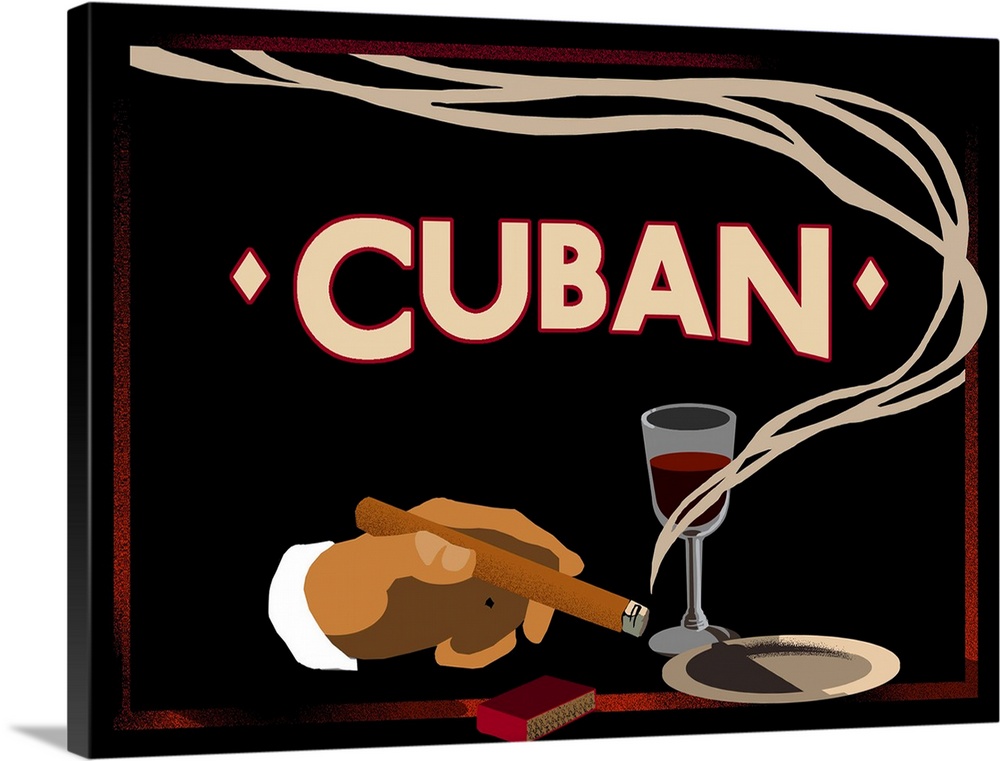The image is a vibrant mock-up of a framed digital graphic with a predominantly black background. At the center of the image, the word "CUBAN" is prominently displayed in an all-caps bold font, outlined in red, flanked by two diamond symbols on each side. In the lower left corner, a hand sporting a white cuff from a shirt or jacket holds a brown cigar, with its smoke elegantly curving up and to the right, weaving over the bold text. Beside the hand is an empty plate and a glass of red wine. A red matchbox and what appears to be an ashtray are also visible in the scene. Surrounding the image is a red band adorned with tiny black dots, and the entire piece is framed in a plain black frame.